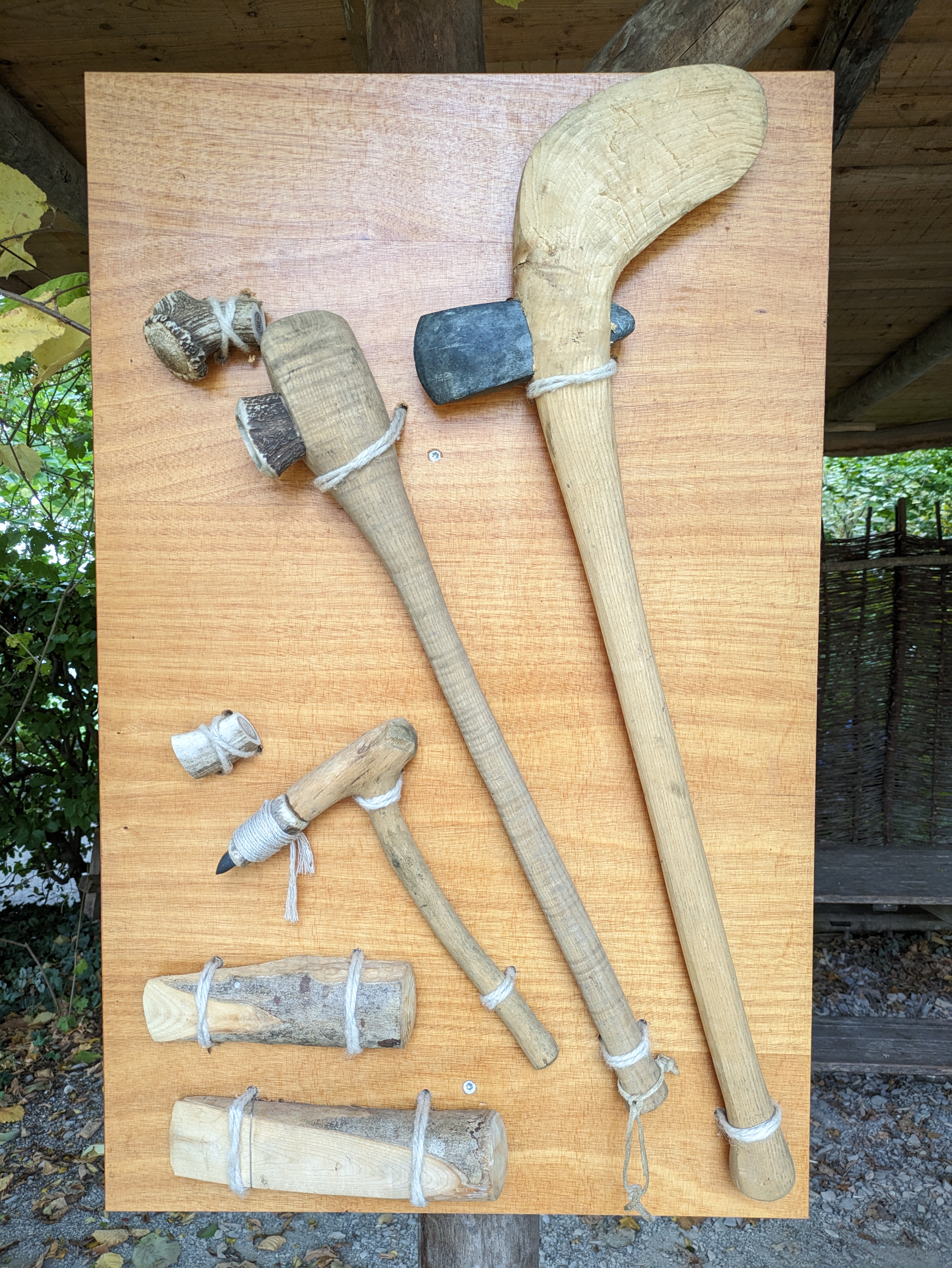The photograph depicts a display of modern recreations of Stone Age tools mounted on a vertically-standing wooden board with a visible wood grain. The tools, crafted from wood and stone, are securely tied to the board using twine cord threaded through holes. The board itself is affixed to a wooden post and is showcased in an area with a wooden ceiling and what appears to be a hut bottom to the right, surrounded by an environment rich with trees, plants, and brown leaves.

The tools vary in size and function, ranging from primitive axes and rudimentary paddles to pointed implements designed for scraping, scratching, pounding, or splitting wood and rock. Notable among them is a tool resembling a short hockey stick with a chipped stone dagger functioning as a primitive axe. Some tools have finely shaved wooden handles, while others feature pointed stone tips, emphasizing their ancient yet functional design. The display also includes wedges or devices at the bottom, likely intended for hammering and splitting materials. The surroundings of the display include greenery on the left side, brown stems, green leaves, and a combination of white and gray rocks on the ground, reflecting a setting that enhances the historical context of the tools.